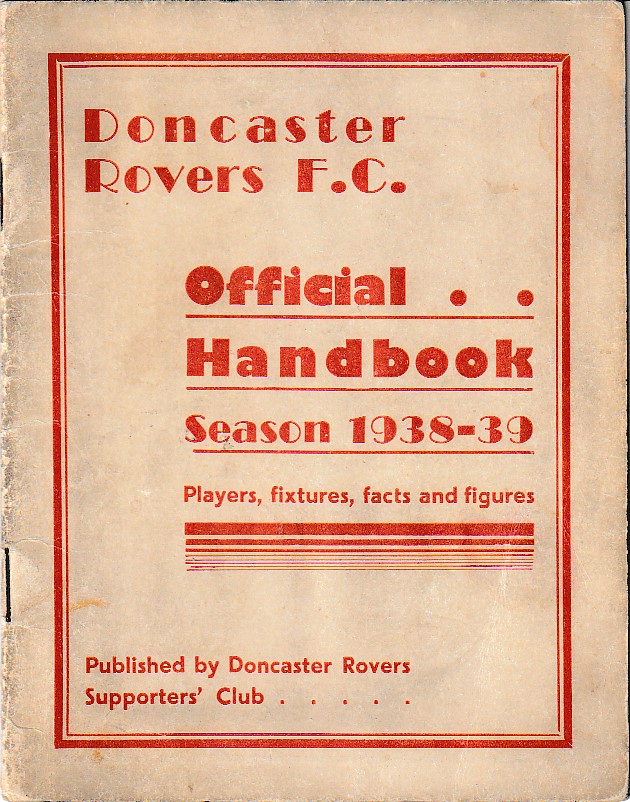The image depicts the official handbook of Doncaster Rovers F.C. for the 1938-39 season. The cover features a vintage cream-colored background with a red border encircling the text. The text, printed in red and using a luxurious font typical for clubs and restaurants of the era, includes "Doncaster Rovers F.C. Official Handbook, Season 1938-39," followed by "Players, Fixtures, Facts, and Figures." Decorative horizontal lines separate this information from the bottom of the cover, which states, "Published by Doncaster Rovers Supporters Club," followed by five dots. The handbook is visibly aged, with heavy wear, crumpling, scratches, and dirt around the edges. Staple marks are evident on the left-hand side, indicating the pages are bound together in this manner.